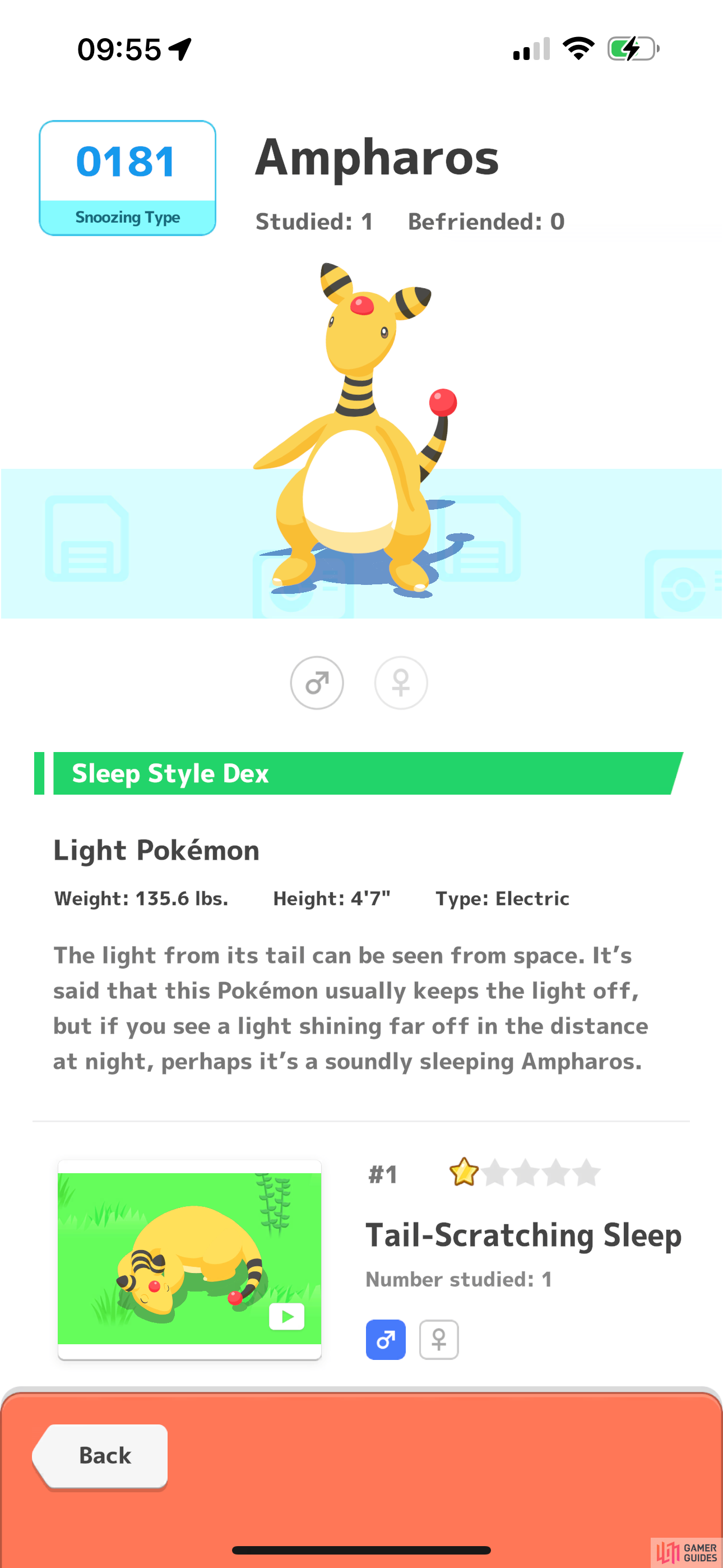In the image, a creature known as Ampharos is depicted. Ampharos is an Electric-type Pokémon, characterized by its distinctive yellow color. Currently, it has been studied but not yet befriended. A number tag labeled "01H1" is visible in the top left corner of the image. Ampharos has a particular snoozing style and enjoys the company of other Pokémon. The creature weighs 135.6 pounds and stands at a height of 4 feet 7 inches. Remarkably, Ampharos possesses a unique tail that can emit light visible from space. Normally, Ampharos keeps its light off, but if you ever see a light shining in the distance at night, it might be a soundly sleeping Ampharos.